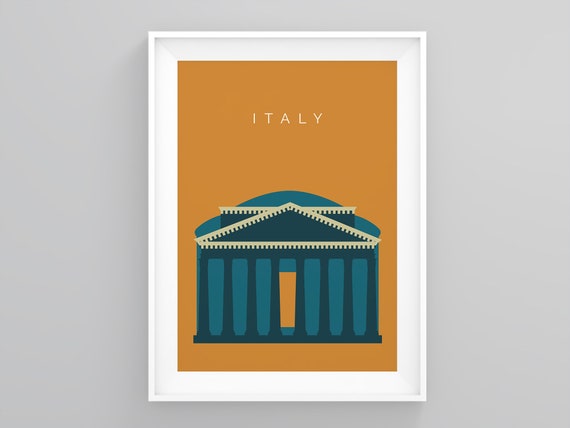This image is a photographic depiction of a framed print, hung indoors on a solid gray to lavender-blue colored wall. The frame is a thick white wood and contains a vertical, rectangular illustration. The upper part of the print features the word "ITALY" in all capital white letters, centered on a dark orange background. Below this text is an illustration of a grand building that replicates Roman architecture, depicted in varying shades of blue. Dominating the lower part of the print, the building has a triangular roof bordered in white and a flat roof behind it. Eight dark blue columns support this structure, with an orange section in the middle suggesting an entrance. The detailed representation of the columns and the building’s facade evoke the elegance of classical architecture.